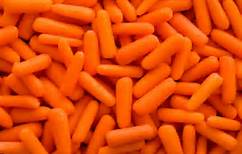This is an indoor, close-up photograph of a bountiful collection of baby carrots, filling the entire frame from top to bottom and left to right. The snackable mini carrots, commonly found pre-cut in the produce section of grocery stores, are approximately two to two and a half inches long and vary in diameter from half an inch to three-quarters of an inch. They exhibit a fresh, beautiful orange hue, though an earlier description inaccurately mentioned them as bright yellow. The carrots are arranged in various orientations—vertical, horizontal, and diagonal—showing some thicker and some pencil-thin. The image is tightly focused and evenly lit, presenting an overhead view that offers no additional visible details beyond the vibrant, ready-to-eat carrots.